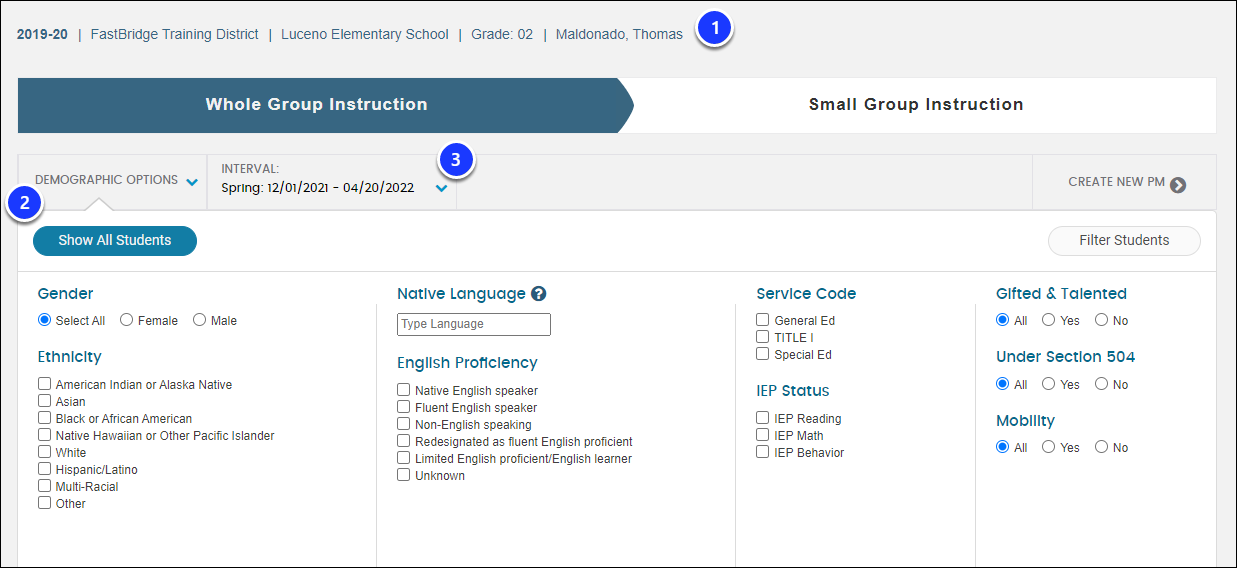This image is a horizontal screenshot of a teacher information panel for the academic year 2019-2020. The teacher's name, Thomas Maldonado, is prominently displayed. 

At the top left corner, the image denotes the specified academic year. There are several sections labeled "Fast Bridge Training District," "Lucerno Elementary School Grade 2," and "Maldonado Thomas," with a circled blue number '1' adjacent to Thomas's name.

Beneath these sections, a choice bar allows for the selection of either "Whole Group Instruction" or "Small Group Instruction," with "Whole Group Instruction" being the current selection. Directly below this bar, a dropdown menu offers various demographic options, accompanied by an interval selection feature. A circled blue number '2' appears next to the demographic options dropdown, and a circled blue number '3' is to the right of the interval selector.

Further down, two buttons labeled "Show All Students" and "Filter Students" provide additional functionality. The lower portion of the image displays categories pertinent to student types, including Gender, Ethnicity, Native Language, English Proficiency Level, Service Code, IEP Status, Gifted and Talented, Section 504, and Mobility. 

All selections within these categories indicate inclusive parameters, as denoted by blue circled indicators for "All Gender," "All Gifted and Talented," "All under Section 504," and "All Mobility."